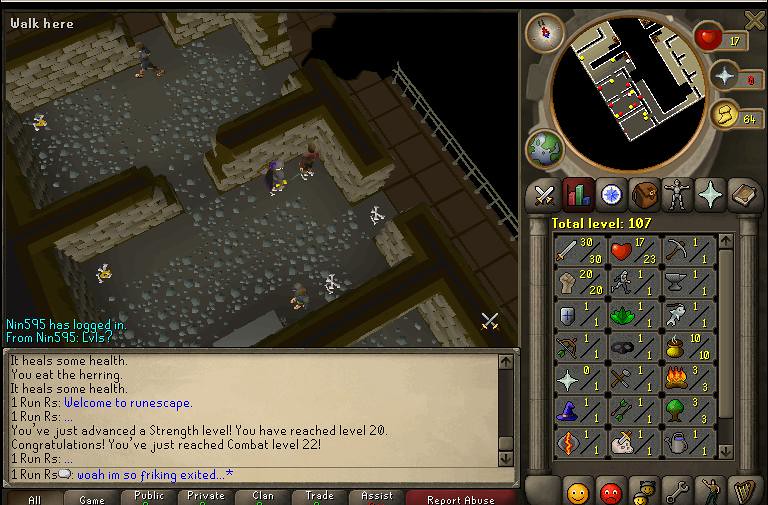This image is a detailed screenshot of an online medieval-themed video game, likely "Runescape." The scene is set in a maze-like environment with gray brick walls and a brown floor, bordered by a gray railing. The user "nin595" is logged in, as indicated by the text in the bottom left. Central to the image is a dialogue box displaying messages such as "it heals some health, you eat the herring," and "you've just advanced a strength level, you have reached 20," celebrating the player reaching combat level 22.

To the right side of the screen, there's an interface that includes a variety of icons and stats: a sword with "30/30" beside it, a heart with "17/23," and other symbols like a shield, a fire, a tree, a pot, a wizard hat, and a wand. Above these icons, the total level is shown as 107. In the bottom right corner, there are emoticons and utility icons including a yellow smiley face, red sad face, a wrench in a square, and two other smiley faces.

Overall, the game interface is rich with details, featuring health meters, an inventory with objects and tools, and clickable icons that direct the player to different parts of the game. The environment depicted appears navigable with little characters on a road, surrounded by sidewalks and fences, suggesting an exploratory or mission-based gameplay experience.